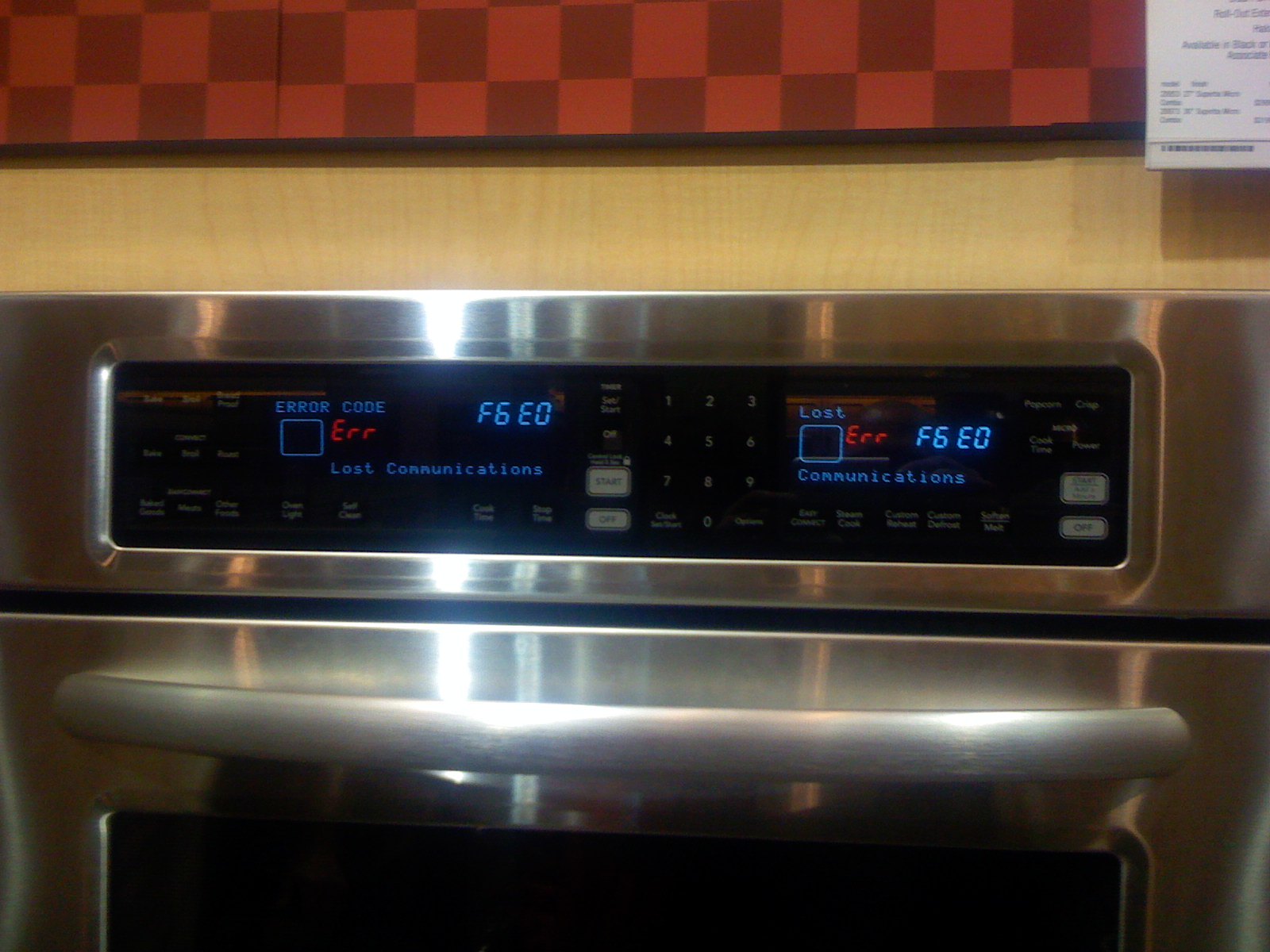This is a close-up photograph of a high-end stainless steel oven embedded in a kitchen wall. The main focus is the oven's control panel, which dominates the central horizontal band of the image. The panel features numerous buttons, including a number pad, start, stop, and off buttons, though many of the smaller text descriptions are difficult to discern due to their size. Prominently displayed on the panel are error codes: "F6EO" in blue and "ERR" in red, accompanied by the message "Lost Communications" also in blue. These error messages appear on both the left and right sides of the control panel, which has a black background framed by a metallic silver border.

Beneath the control panel, a large, sleek silver handle spans horizontally, slightly curved outward, suggesting it is the oven door handle. Below this handle is a dark, square glass window that provides a glimpse into the oven's interior.

The oven is set against a light brown wooden wall, contributing to the kitchen's warm ambiance. Above this, a decorative strip of light and dark red checkered pattern adds a splash of color to the scene. In the top right corner of the image, a piece of white paper with unreadable black text is pinned or taped to the wall. The photograph appears slightly blurry, with some light reflecting off the shiny metallic surfaces, indicating the need for a quick camera wipe.